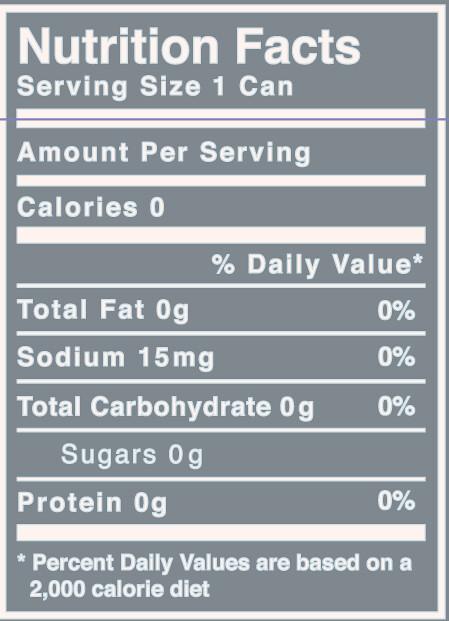This image showcases a detailed Nutrition Facts label, presented in a concise and organized manner. The label features a dark gray background and is framed by both a dark gray outer outline and a subsequent white outline. All text on the label is rendered in white, ensuring high contrast and readability against the dark gray backdrop.

At the top of the label, bold white text reads "Nutrition Facts." Directly below this heading, the serving size is specified as "one can." A prominent white bar demarcates this section from the next.

Following the serving size, the label indicates the "Amount Per Serving," separated by another white bar. The caloric information is highlighted next, with the word "Calories" and the number "0" presented, again set apart by a white bar.

The lower portion of the label breaks down the percent daily values of key nutritional elements, including total fat, sodium, total carbohydrates, and protein. Each nutrient is listed with its respective percentage, providing a clear overview of the nutritional content.

At the bottom of the Nutrition Facts label, an asterisk leads to a footnote that states, "Percent Daily Values are based on a 2000 calorie diet," offering important context for the provided nutritional percentages. This detailed and clear label serves to inform consumers about the nutritional aspects of the product inside, although the actual product to which the label is affixed is not visible in the image.